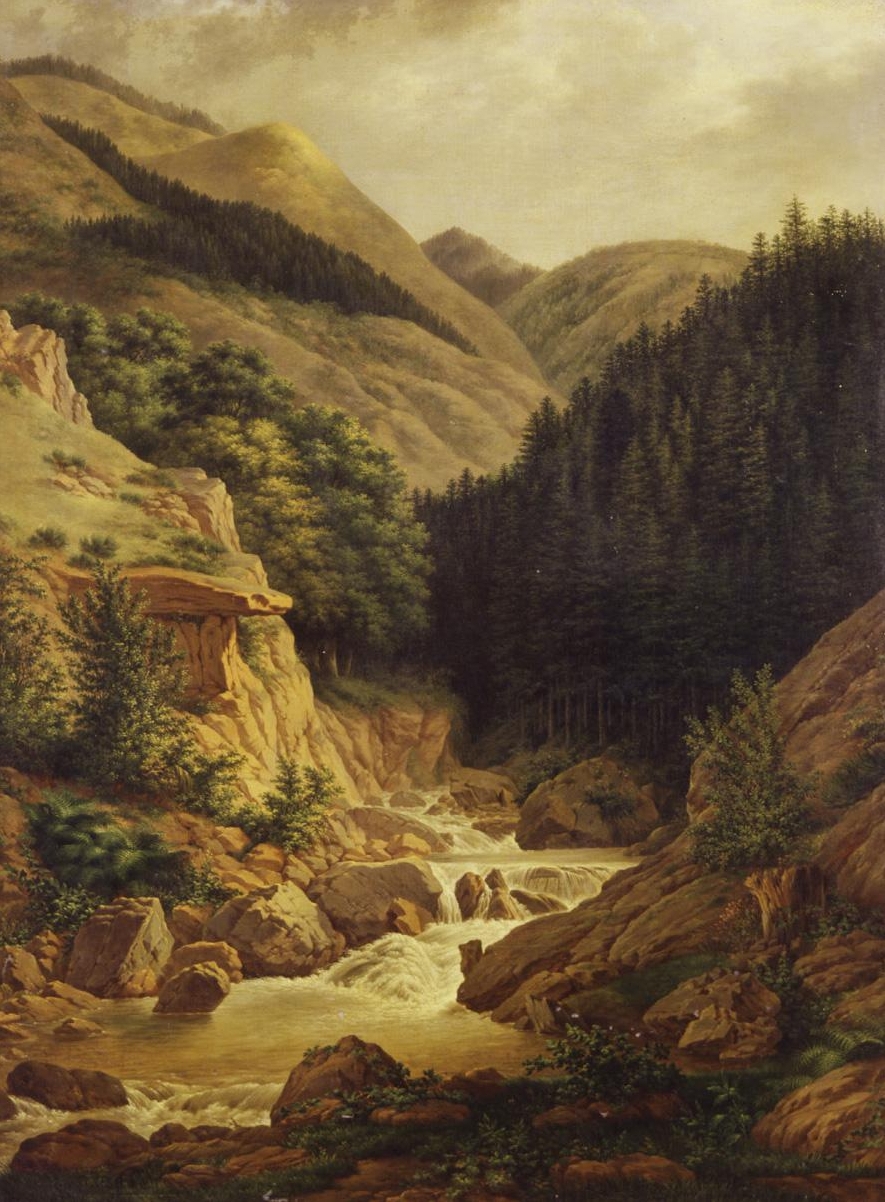This painting vividly captures a serene and dynamic natural landscape. At the forefront, a river, adorned with rapids and cascading white water, originates at the midground and advances towards the viewer, weaving around boulders and rocks. Flanking the stream, green shrubbery and ferns thrive on rocky inclines, with mossy plants clinging to the stones. To the left, a collection of small plants sprouts, enhancing the lushness of the scene. In the background, thick forests of evergreen trees rise, primarily to the left and right, contrasted by rolling hills—some grass-covered and others with a smattering of brown hues. These hills give way to the tableau of the expansive sky, which is a mix of cloudy gray and dull yellow tones, casting an overcast ambiance over the entire landscape. With its interplay of soft browns, greens, and the occasional rusty tinge, the painting exudes a soft, almost dreamlike quality, encapsulating the tranquil yet powerful essence of nature.